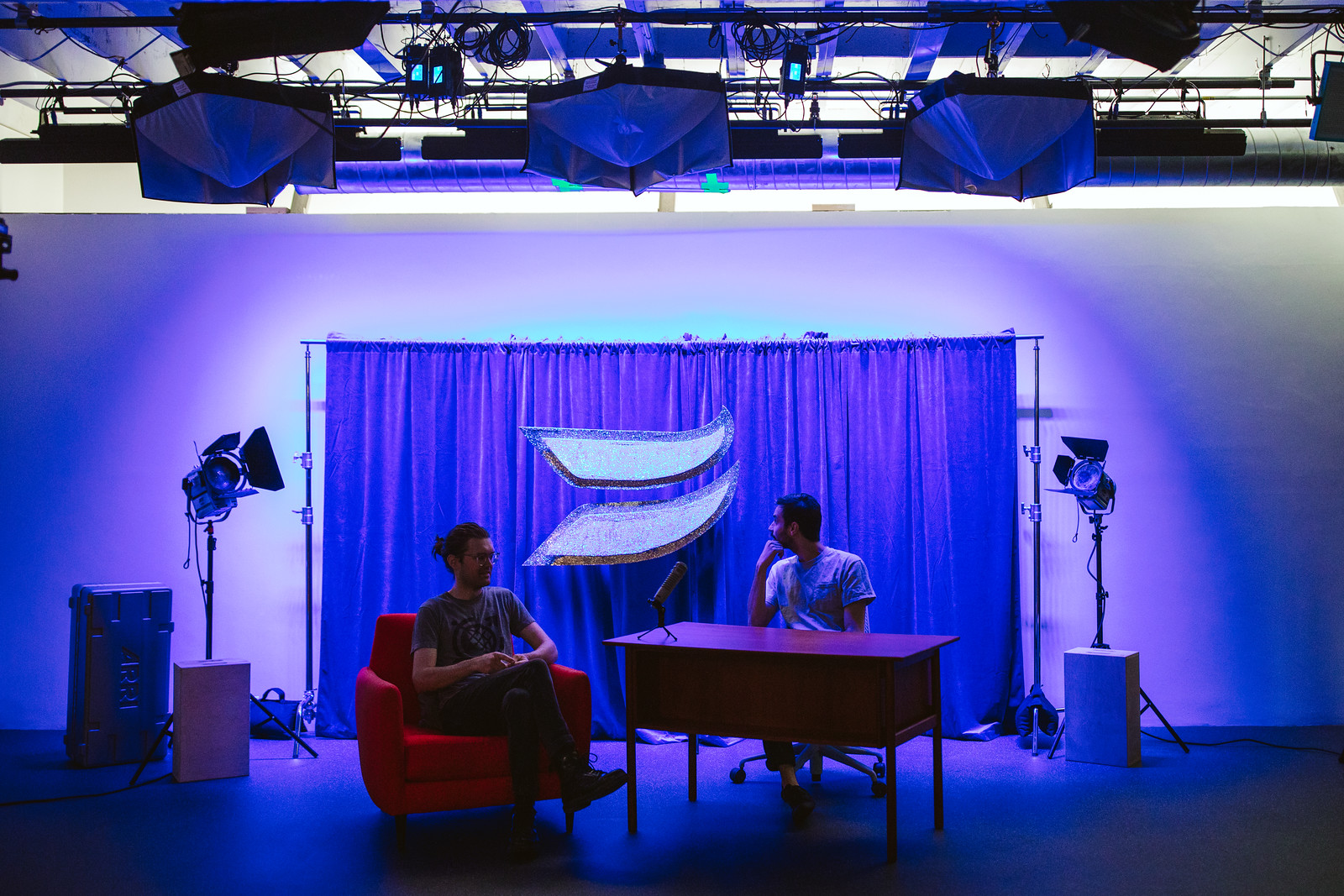The image depicts the interior of a set designed to resemble a talk show. At the center, there is a man with short brown hair seated behind a desk with a microphone mounted on it, wearing a blue tee. To his side, a man with brown hair tied in a bun, dressed in a gray T-shirt and dark pants, sits comfortably in a red easy chair. The backdrop consists of a blue curtain hung on a rail, with lighting equipment in front of it, potentially used to reflect and diffuse light. The ceiling reveals a very industrial look with lights and wires mounted on a metallic framework, including a catwalk. Additionally, there are spotlights and other lamps highlight the scene, creating a well-lit environment. To the left of the setup, a storage chest likely used for hauling equipment is visible, adding practicality to the otherwise clean and organized set.